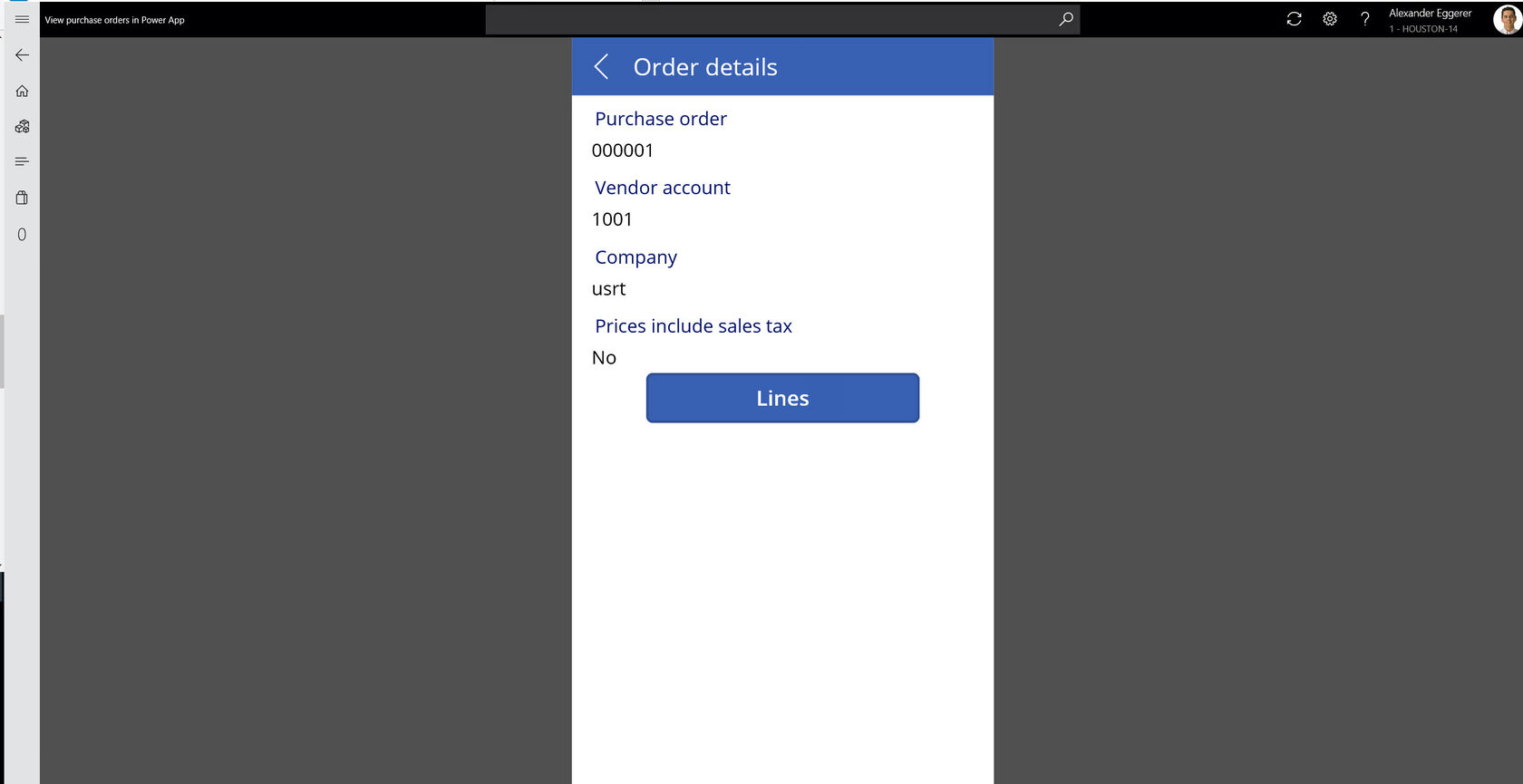Screenshot of a gray computer screen with a charcoal gray background. The screen contents are partially obscured, making it difficult to identify the exact context. In the upper right corner, there's a small image of an individual, potentially indicating the user's profile, along with an unclear name.

Dominating the center of the screen is a prominent pop-up window titled "Order Details." This title is displayed in white text on a blue banner. Below the banner, the pop-up contains several fields presented in black font with mixed capitalization:

1. **Purchase Order**: 000001
2. **Vendor Account**: 10001
3. **Company**: usrt (in lowercase letters)

Additionally, the pop-up indicates that prices do **not** include sales tax. At the bottom of the pop-up is a blue button with white text, although the exact wording is not discernible.

The user appears to be in the process of viewing or managing an order, with interactive elements suggesting the ability to navigate or perform actions related to the order details.